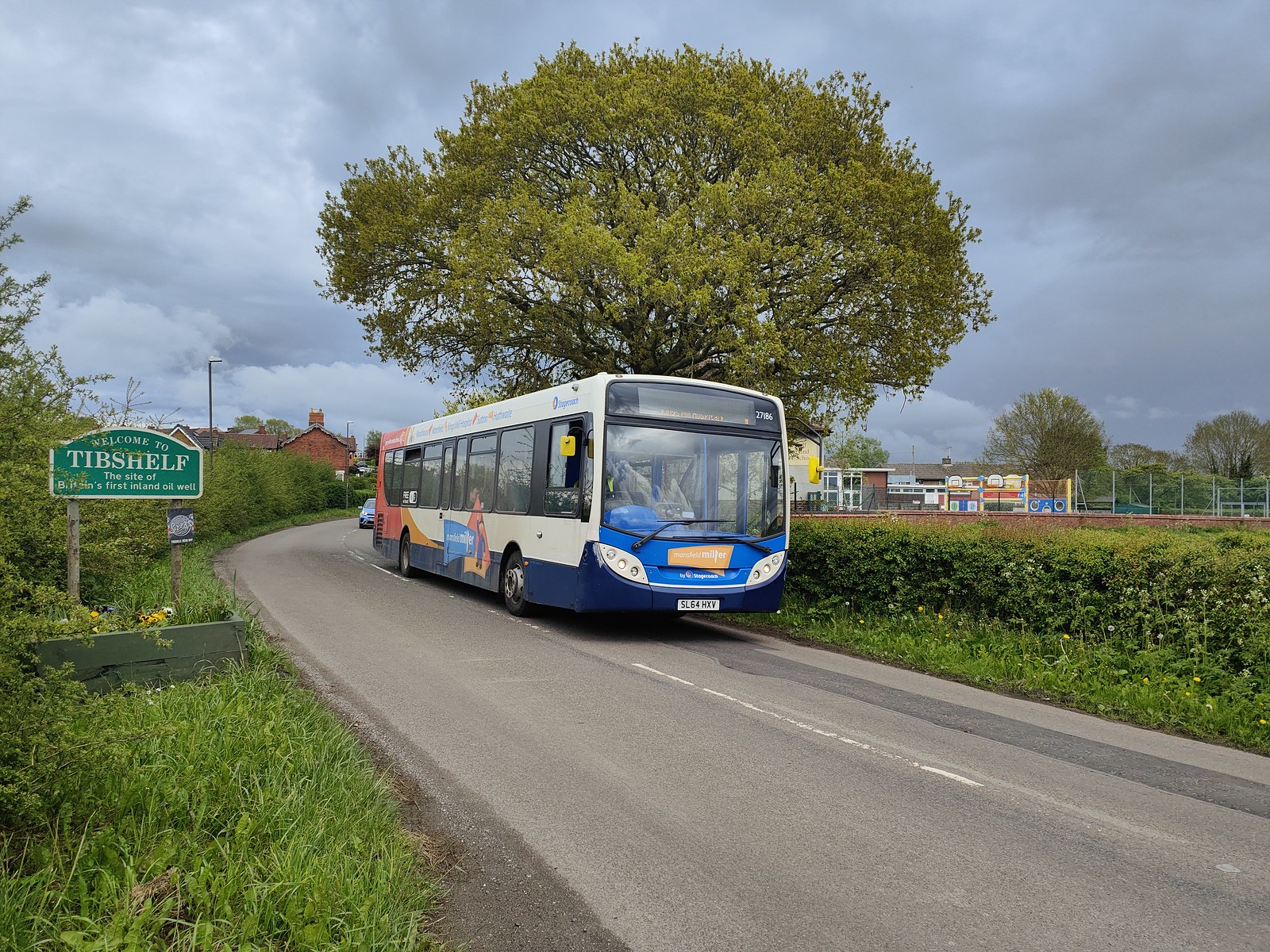This photograph captures a vibrant outdoor scene in Tibshelf, England, featuring a prominently placed blue and white public transit bus with an orangish-reddish design on its rear, traveling down a rural road. The roadway is flanked by lush grass and various bushes, adding a vivid green contrast to the image. Towering behind the bus is a large, bushy tree with green leaves, set against a backdrop of overcast skies filled with gray clouds, hinting at a potential storm. On the left side of the road, there's a green historical sign that reads: "Welcome to Tibshelf, the site of Britain's first inland oil well," in white text. The right background reveals what appears to be a brightly colored playground or perhaps a sports field, indicated by visible equipment such as basketball hoops. A red-bricked building with a chimney and a streetlight peek through on the left side, while a largely obscured car follows the bus. This detailed depiction suggests a serene, quiet community scene with a mix of natural and man-made elements.